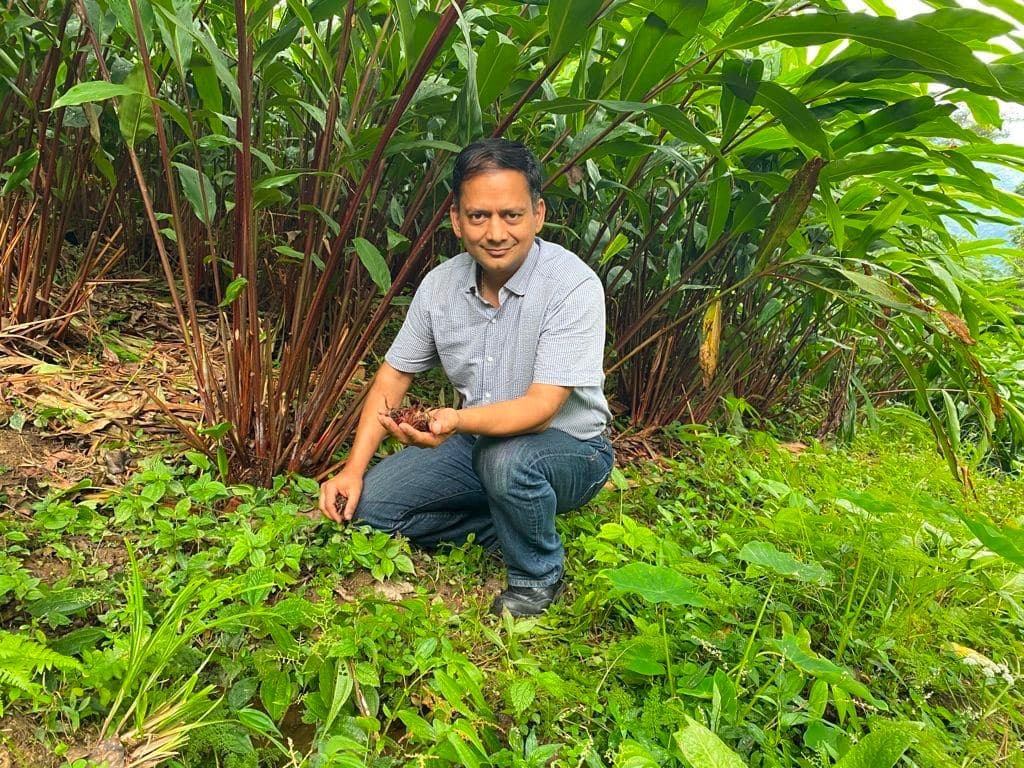In this photograph, a man is captured kneeling outdoors amidst a lush, green environment. He is wearing a light blue, short-sleeve button-up shirt paired with blue denim jeans and black leather shoes. The setting is a mixed terrain of green and brown, with dense green foliage and some brown leaves or dirt visible on his left (the viewer’s right). Towering behind him is a prominent plant with long, broad leaves resembling those of a coconut tree, contributing to the rich greenery around. The man is facing the camera with a proud smile, showcasing something he holds in his left hand—possibly a large bug or an interesting plant. In the distance, a hill can be vaguely seen, adding depth to the scene. Remarkably, despite the abundance of plants, there are no visible flowers in the vicinity.